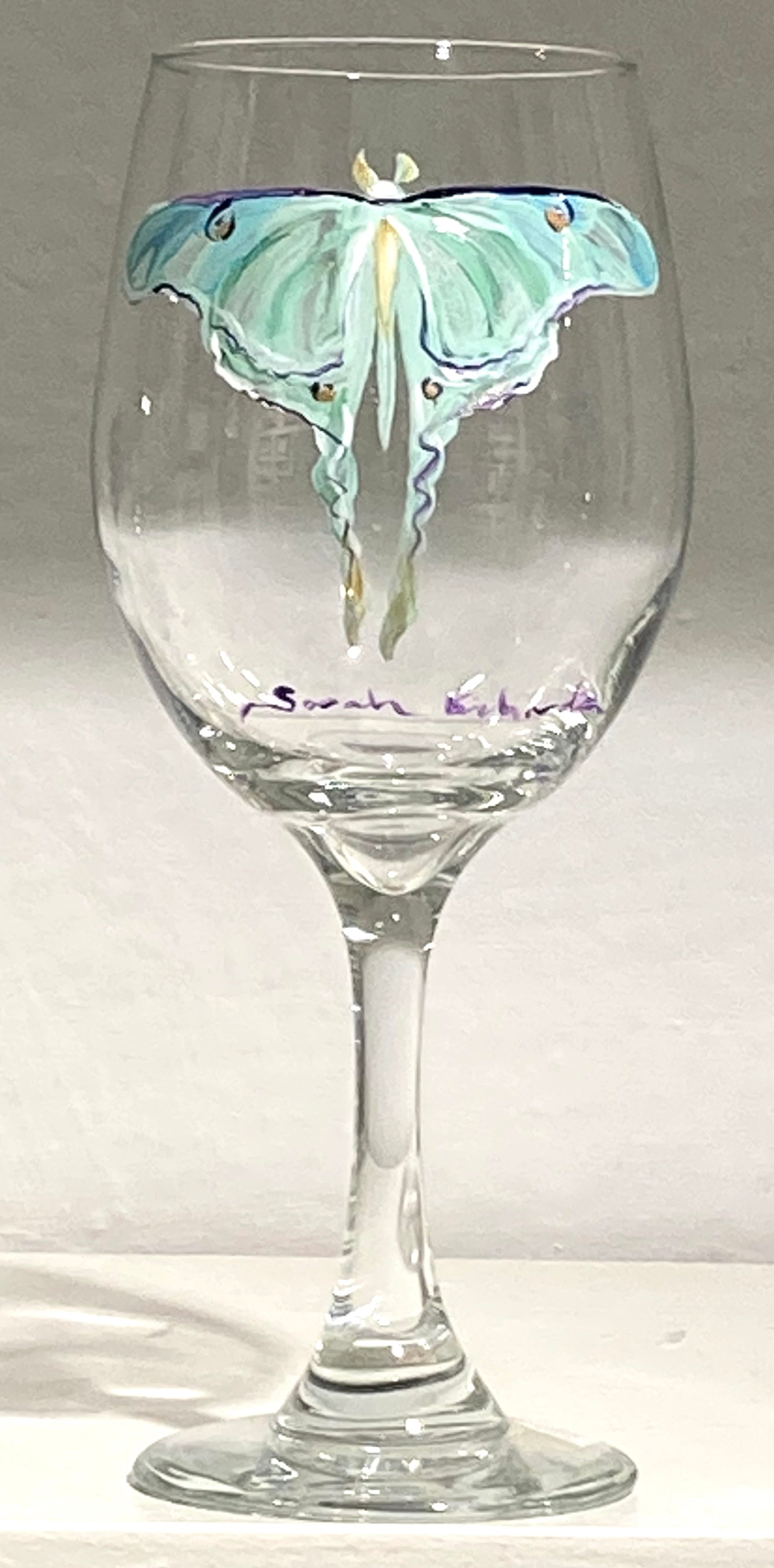This photograph captures a tall, long-stemmed wine glass positioned on a white surface with a white wall in the background. The glass is empty but is distinguished by a beautifully painted butterfly or possibly a moth on one side. The wings of this creature exhibit a captivating gradient of colors, ranging from shades of blue and green to a vibrant turquoise. Accentuating the wings are dark purple designs and subtle orange dots, some of which are outlined in purple. Notably, the wings extend into two zigzag tails with a dull golden-brown hue. Beneath the butterfly, a signature in purple cursive letters reads "Sarah," though the last name remains unclear. The butterfly's head and outstretched wings, combined with the elegant signature, lend the glass a uniquely artistic and personalized touch.